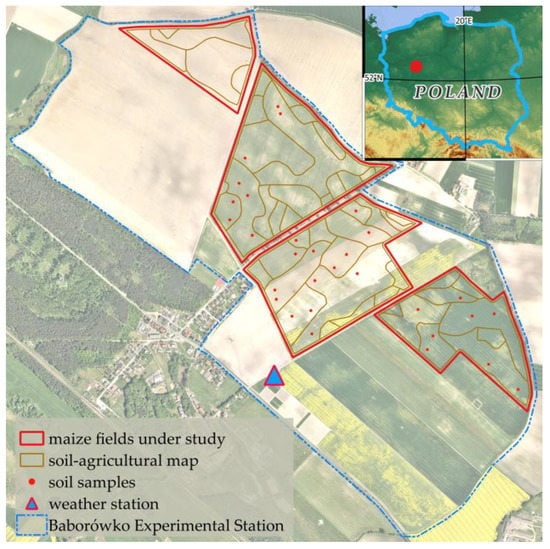This image is a detailed agricultural map highlighting different features and research areas within Poland. The top right corner includes a smaller inset map of Poland with a blue outline and a red circle on the top left side of this inset, pinpointing the broader region of study. The main map is predominantly colored in white, green, and gray with several blue and red outlines marking various areas and fields.

The map's legend is located at the bottom left corner and is essential for understanding the annotations. According to the legend:
- A red outline denotes maize fields under study.
- A gold outline signifies the soil agricultural map.
- Red circles correspond to soil sample locations.
- A blue triangle with a red border represents a weather station.
- A dotted blue border designates the Babaro Co. Experimental Station.

The main map includes various outlined areas: fields outlined in dotted blue to indicate experimental stations, and several red outlines marking specific maize fields under study. There are also multiple red circles showing soil sampling sites. The map seems to capture not just the layout of agricultural activities but also includes a topographical representation of a small city and surrounding rural areas.

Overall, this detailed caption captures the map's purpose of showcasing agricultural research and the locations of different experimental activities within Poland, aided by a comprehensive legend and various colored outlines marking key areas of interest.